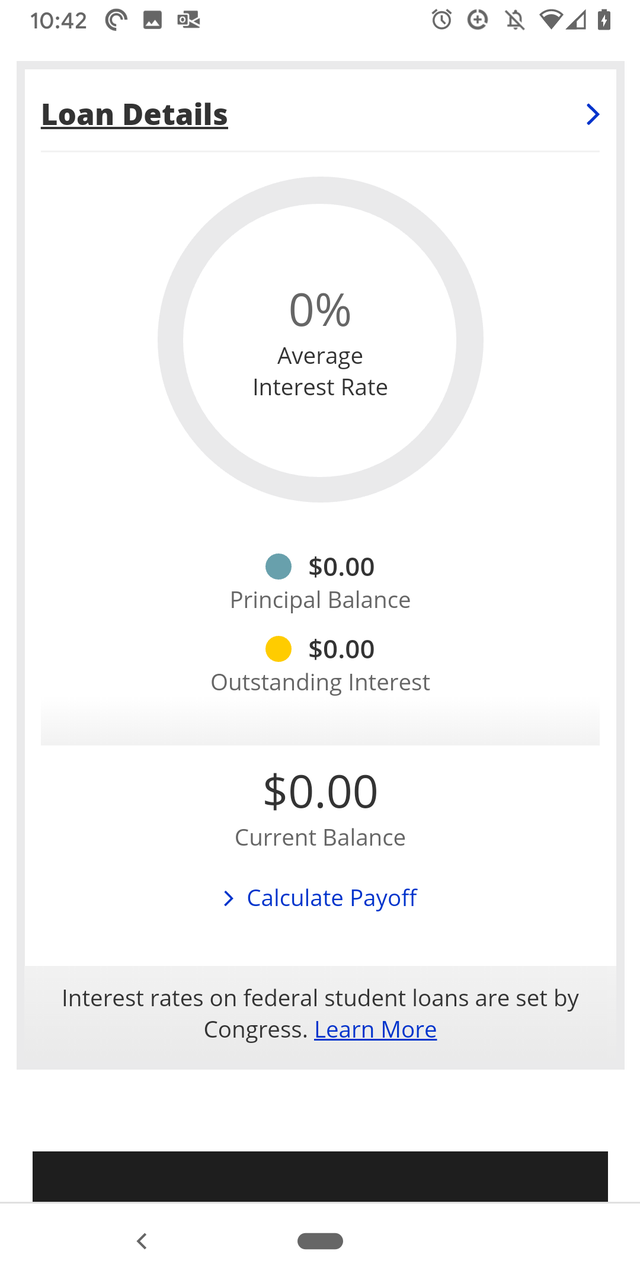This is a detailed screenshot of a smartphone application interface. The top-left corner displays the current time as 10:42, alongside various icons indicating Outlook notifications, an alarm, and a silence mode. Below these icons, the central section of the screen focuses on loan information. The loan summary shows an average interest rate of 0%, a principal balance of $0 (highlighted with a blue circle), and an outstanding interest of $0 (marked with a yellow circle), culminating in a current balance of $0.

A prominent blue button labeled "Calculate Payoff" is positioned below these loan details. A note below this button informs users that interest rates on federal student loans are determined by Congress and includes a blue "Learn More" link for further information. The entire interface features a clean design with a white background and primarily black text, except for the clickable blue links. 

Additionally, there is a "View Loan Details" blue button adjacent to the loan summary, which users can click to see more detailed information about the loan. In summary, this screenshot captures an app that shows a user’s loan at 0% interest and a $0 balance in a neatly organized and intuitive layout.